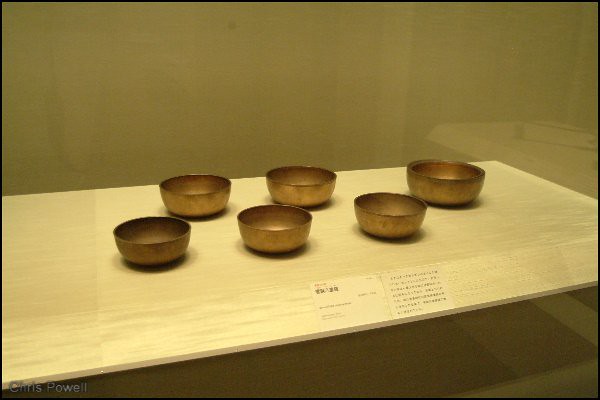The image depicts a shelf, likely in a store or museum, holding six small, circular bowls arranged in two staggered rows. The shelf, crafted from light-colored wood, supports bowls that exhibit a medium brown to brassy, coppery gold hue. The front row consists of three bowls, with another three behind them, all neatly aligned in a staggered formation. One of the bowls stands out due to its slight size difference, appearing thicker and a bit taller than the others. A price tag and a paragraph of text, though blurred and unreadable, accompany the display on the shelf's front, hinting at an informative or descriptive purpose. Reflecting potential protective glass, the background is a dark beige color. Additionally, there are two white pieces of paper that likely explain the exhibit, and in the lower left corner, the name "Chris Powell" is inscribed in white letters. The interior of the bowls reveals a slightly lighter gold color, attesting to their thick, decorative, possibly copper material. The overall scene evokes a sense of historical artifact presentation, perhaps echoing the aesthetic of a museum exhibit.